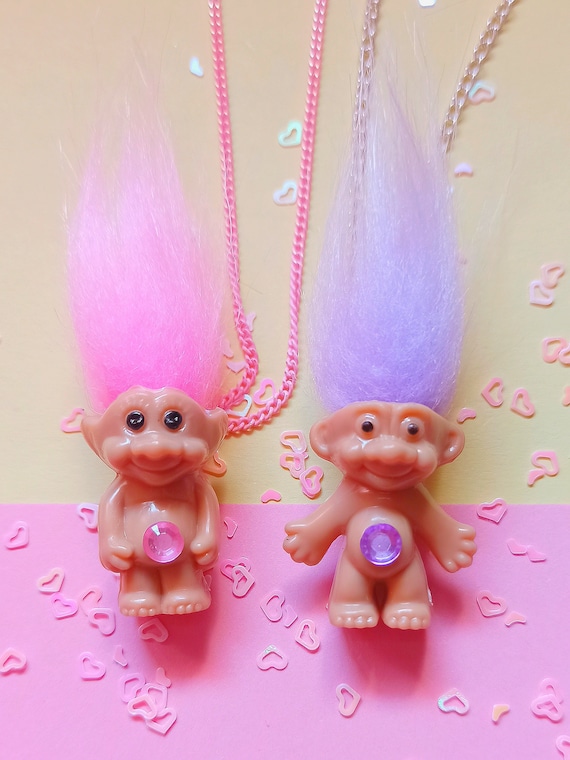This is a color photograph of two troll dolls, set against a background that is tan in the top two-thirds and pink in the bottom third, adorned with scattered, metallic, iridescent pink hearts. The troll doll on the left features tall, bright pink fuzzy hair, and a peach skin tone body with large earlobes. It has a pink gem where its belly button would be and is attached to a long, pink metallic chain, suggesting it could be worn as a necklace. The doll's hands are resting at its sides. The troll doll on the right is identical in design but sports purple fuzzy hair and a matching purple gem belly button. This doll has its arms outstretched, seeming to welcome with a smile. Both dolls have large eyes, with the left one displaying eyelashes, adding a delicate touch to their whimsical appearance.